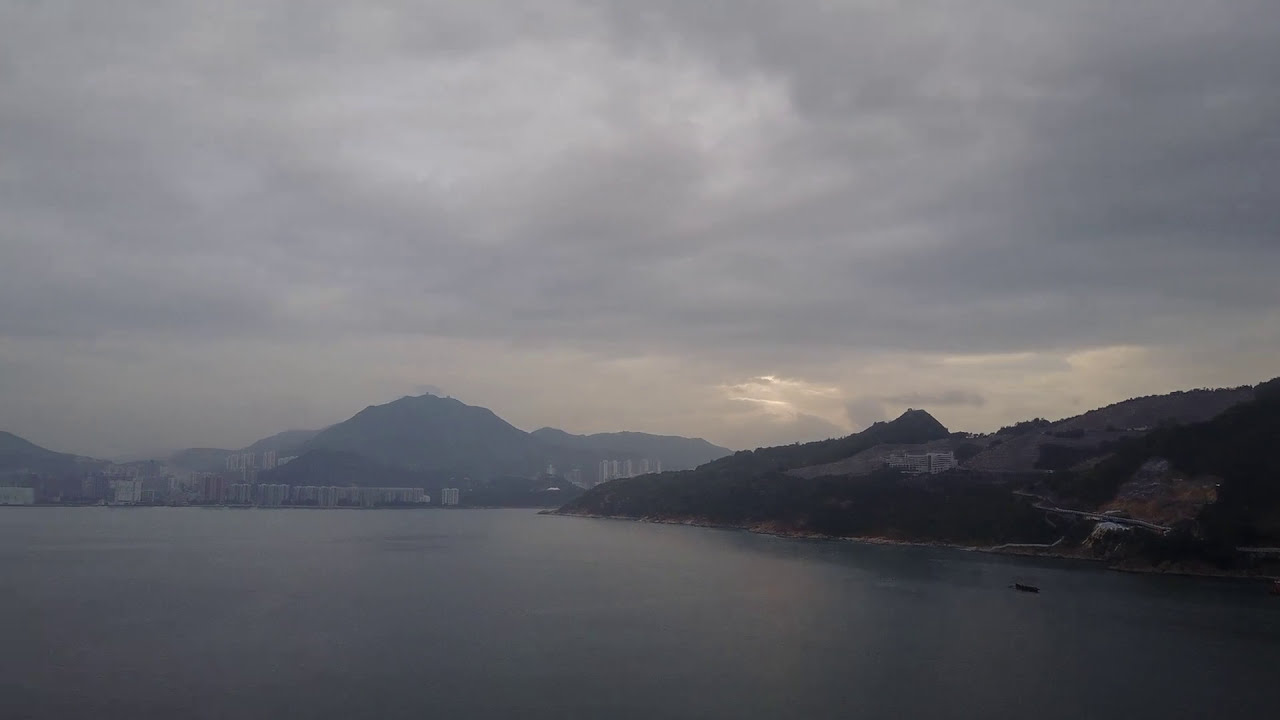The image captures a dreary, overcast evening with a sky dominated by thick, gray clouds, which occupy 60-70% of the frame. The sun, mostly obscured by the clouds, casts a faint, almost imperceptible light from the upper right center of the image. The scene is set against a backdrop of rolling hills that extend from the right side to the distant background. The hills frame a large body of water, which occupies the foreground and appears in a grayish-blue hue, mirroring the somber tones of the sky. Along the shoreline, particularly on the left side, there are scattered buildings and structures. On the right, there is possibly a small boat or object on the water, though it's difficult to discern due to the overall haze. Despite the rugged, rocky shoreline that appears quite elevated from the water, the landscape exudes a sense of untouched wilderness. The light breaking through the clouds in the far distance suggests a fleeting hint of a setting sun, adding a subtle contrast to the otherwise monochromatic and gloomy scene.